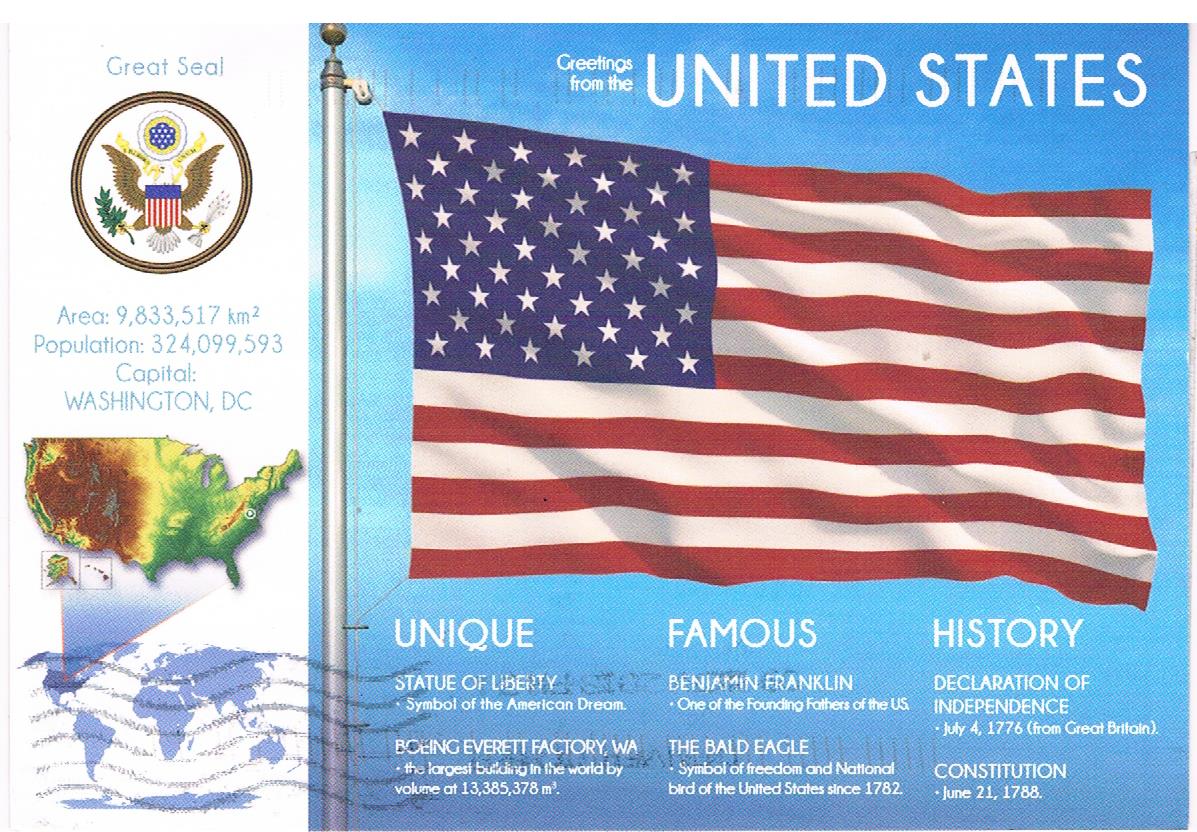This detailed horizontal rectangular postcard prominently features elements representing the United States. On the left side, set against a white background, is the Great Seal of the United States. The seal includes a bald eagle clutching an olive branch in one talon and arrows in the other, surrounded by concentric brown and white rings, with white stars forming a hexagonal pattern. Below the seal, there is a snapshot of geographic information: "Area: 9,833,517 km²" and "Population: 324,999,593." Beneath this, a detailed relief map of the United States highlights the mountainous terrain in the west alongside smaller inset maps of Alaska and the Hawaiian Islands. Additionally, there is a global map indicating the United States' position on the North American continent.

To the right, the background switches to blue featuring a silver pole with the American flag billowing. Above the flag in small white letters are the words "Greetings from the," followed by large white letters spelling out "UNITED STATES." Below the flag, three columns provide historical and cultural information:

1. Unique: "Statue of Liberty, symbol of America's dream," "Boeing Everett Factory (Largest building in the world by volume)," with figures highlighting its vast size.
2. Famous: "Benjamin Franklin," noted as one of the Founding Fathers, and "Bald eagle, symbol of freedom and national bird of the United States since 1782."
3. History: Mentions key historical documents, "Declaration of Independence, July 4th, 1776 (from Great Britain)" and "Constitution, June 21st, 1788."

This image quintessentially captures the patriotic spirit and significant historical milestones of the United States, making it a detailed and illustrative representation.